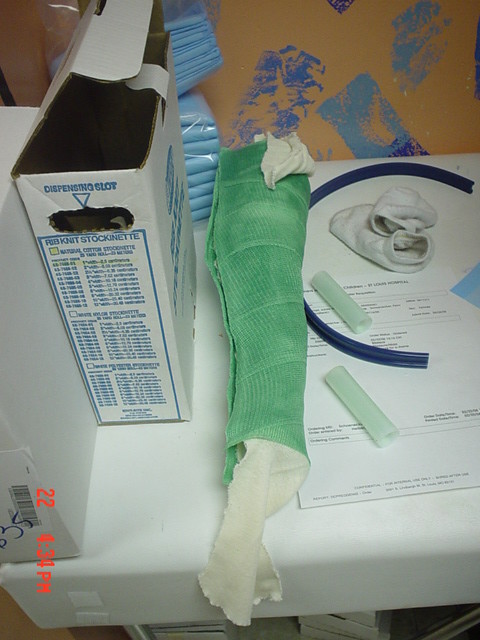The image depicts what appears to be a medical table holding various items, likely in a clinical or unfinished basement setting. Central to the scene is a mint green cast that has been cut open, revealing white lining protruding from both ends, suggestive of its recent removal. Alongside the cast lies blue tubing, aligning to the right, and a white box to the left. The table is cluttered with additional medical supplies and items such as folded blue towels or cloths in plastic packets, a cut-up blue tube, and two white socks. Prominently displayed on the table is a piece of paper that possibly includes an invoice or instructions, adding to the clinical nature of the setup.

In the background, the wall, either brown or unfinished drywall, shows various blue paint swatches indicating ongoing renovations or tests of color choices. There is a yellow section of the wall with a specific blue paint mark labeled "22-4-34 PM" in red, suggesting some form of testing or note-taking. The overall impression is one of a workspace in progress, caught in the midst of transition or practical use. The photograph is taken from a downward angle, focusing on the central green cast and associated medical instruments, providing a detailed look at the scene on a white counter space or table.